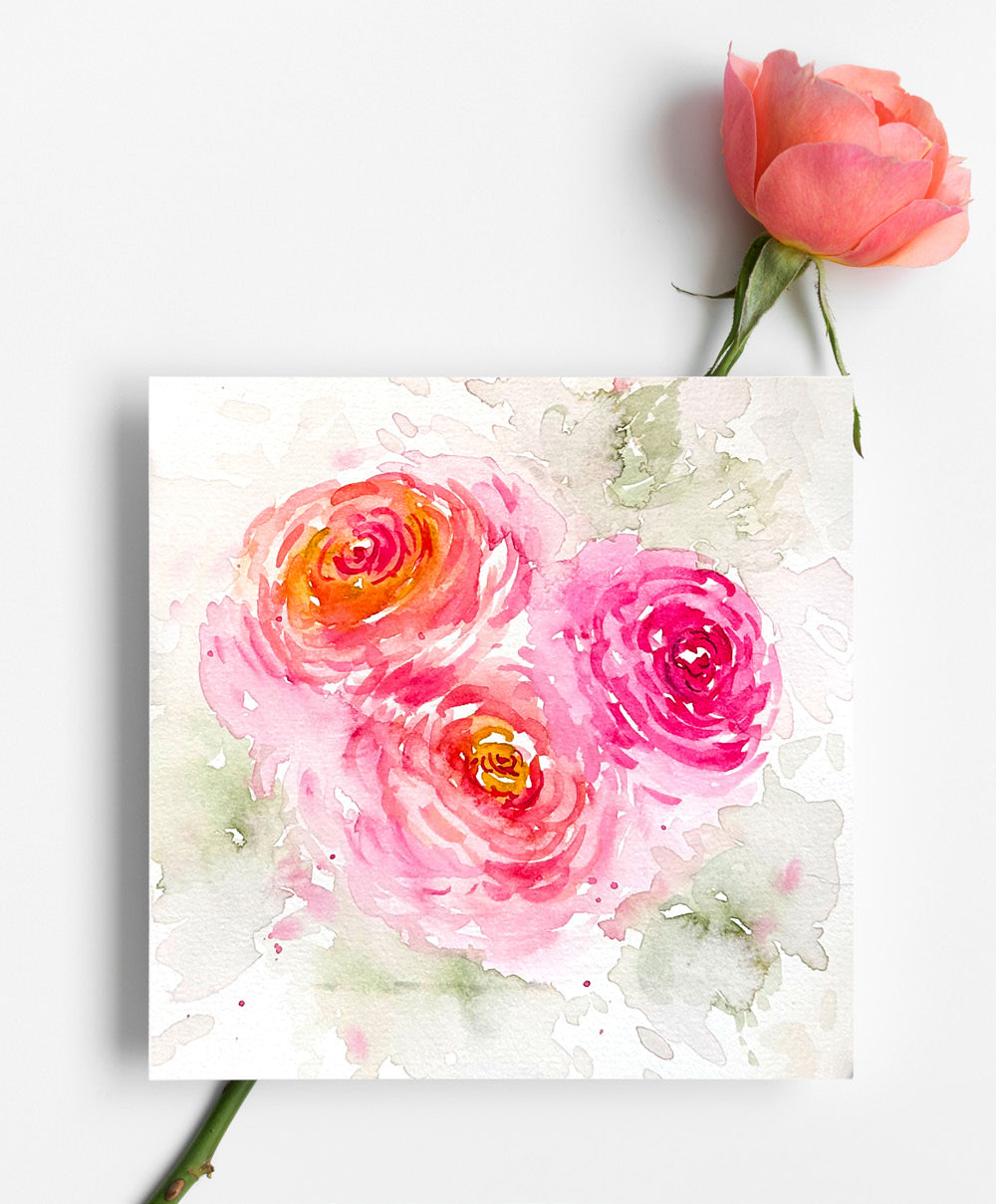In this well-lit studio shot, a small, square watercolor painting is placed on top of a real pink rose, both isolated against a white background or countertop. The painting, approximately 6 to 8 inches on each side, depicts three roses rendered in a loose, impressionistic style. The flowers are painted in shades of pink with orange highlights at their centers, surrounded by pale green splotches that suggest foliage. Beneath the artwork, the natural pink bloom of the rose, accompanied by its long, green, thorny stem, is clearly visible. The image creates a layered effect of painted and real flowers, showcasing the delicate beauty of both mediums. There is no text within the image.